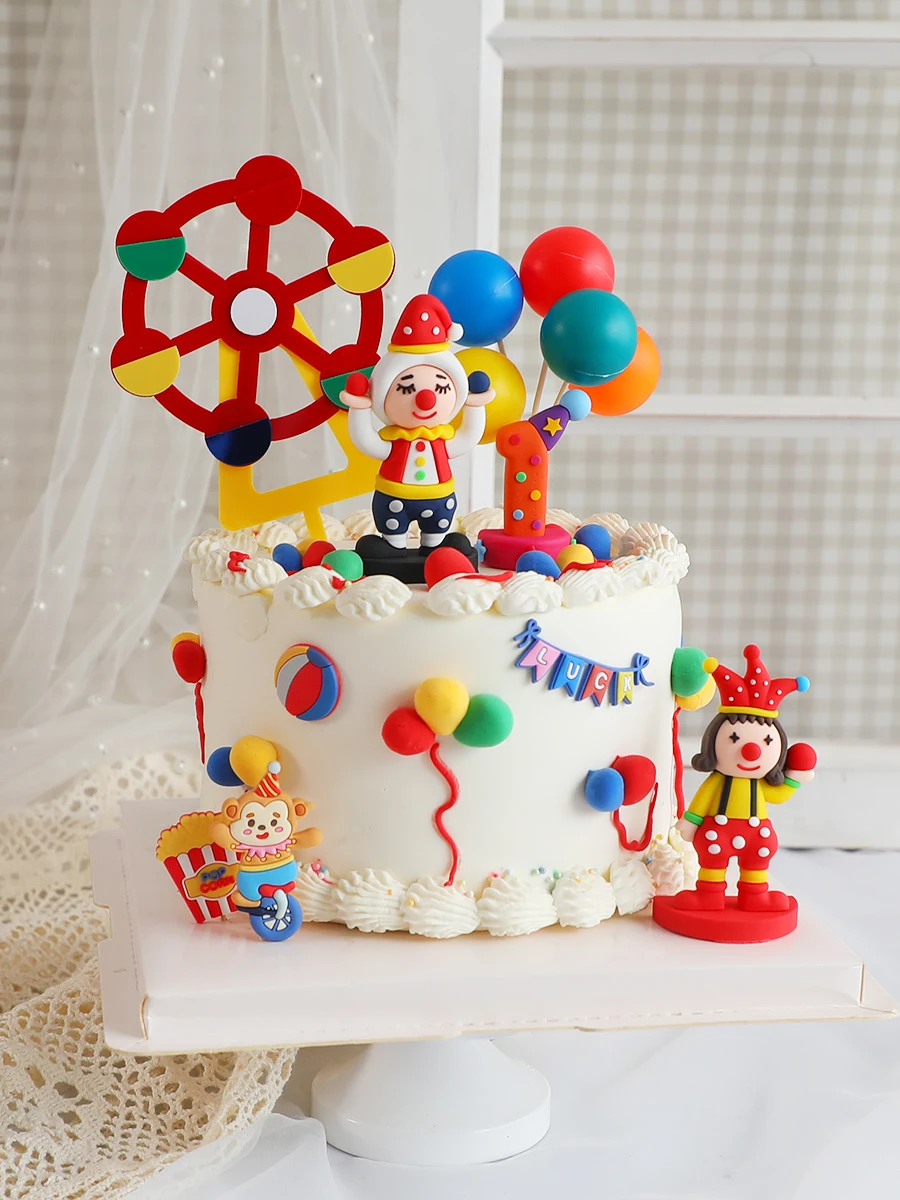This professional, single-layer cylindrical birthday cake is adorned with a smooth layer of white frosting. The top is decorated with an intricate wave-like piping of white icing, which is also present around the bottom edge. Standing prominently on the cake is a festive clown figure and an orange number one topped with a purple wizard's hat, complete with a yellow star and a small blue ball at the tip. Surrounding them are colorful balloons—yellow, blue, red, green, and orange ones—that add to the vibrant scene. 

On the side of the cake, a ribbon spells out the word "luck" in cheerful letters, accompanied by small, colorful flags in pink, blue, red, and yellow. Enhancing the playful theme, a miniature Ferris wheel structure, resembling a merry-go-round, showcases red and yellow balls. The cake also features a whimsical monkey riding a unicycle with a popcorn box on its back and another clown figurine dressed in overalls. 

Set against a white curtain backdrop, possibly near a window, the cake sits elegantly on a white stand with unique shelves and a lace tablecloth underneath, completing the delightful display.